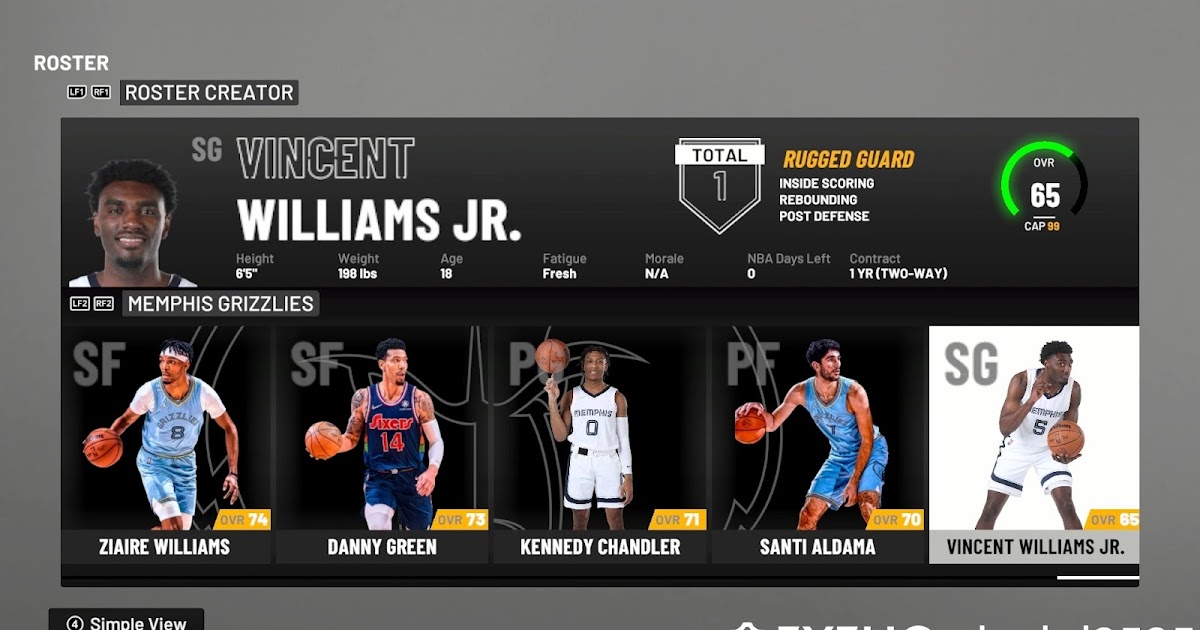Screenshot from NBA 2K Game's Roster Tab: Detailed View of Vincent Williams Jr.

This image is a detailed screenshot from the roster tab of an NBA 2K video game. The top left corner of the screen prominently displays the word "ROSTER," indicating the current section of the game. The focus is on Vincent Williams Jr., whose player profile is shown in detail.

On the left side of the screen is a picture of Vincent Williams Jr. To the right of his picture, his name is displayed in large bold font, and beneath his name, additional information is provided in smaller text. This includes key player statistics such as height, weight, age, fatigue level, morale, remaining NBA days, and contract details. 

The screenshot also highlights Vincent Williams Jr.'s abilities as a "rugged guard," emphasizing his inside scoring, rebounding, and post-defense skills. His overall player rating is shown on the far right, marked as 65.

Below Vincent Williams Jr.'s information, the roster lists other players available for selection, including Zyree Williams, Danny Green, Kennedy Chandler, and Santi Aldama. This indicates multiple roster options within the game.

Overall, the image provides an in-depth look at Vincent Williams Jr.'s profile within the NBA 2K game, showcasing both his individual stats and role-specific attributes.